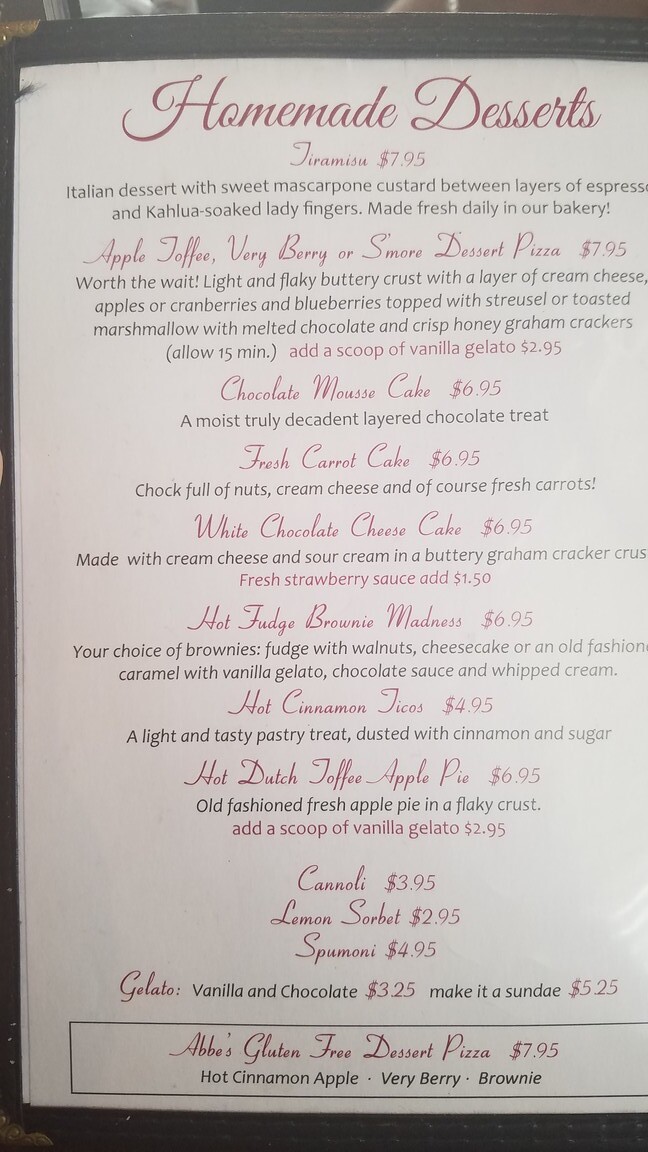The photograph captures a single page of a restaurant menu elegantly presented within a black folder against a white background. At the top, the heading "Homemade Desserts" is prominently displayed in bold red letters. The menu items are listed in red cursive, each accompanied by a detailed description in black text. The mouth-watering dessert options include:

- Tiramisu
- Carrot Cake
- White Chocolate Cheesecake
- Hot Cinnamon (undisclosed item)
- Hot Dutch Toffee Apple Pie
- Abby's Gluten-Free Dessert Pizza

Additionally, the menu features offerings such as gelato, sundaes, cannolis, and sorbets. The surface on which the menu rests is indistinct, making it unclear if it is a tabletop or another type of surface.